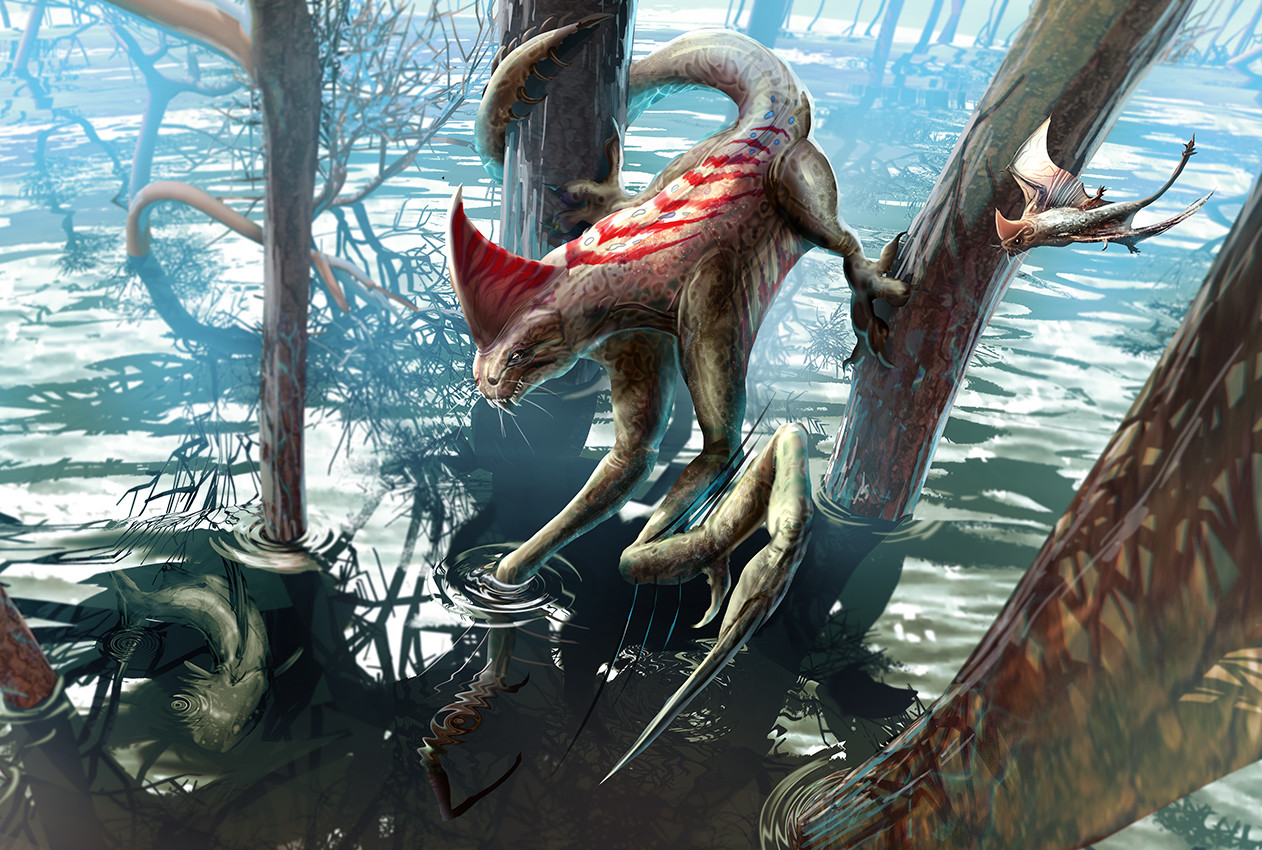The digital illustration depicts an astonishingly unique creature in a mystical, swampy environment. This fantastical beast appears to be a hybrid of several animals, initially resembling a cat but featuring an iguana-like tail wrapped around a submerged tree trunk. With a crimson shark-like fin crowning its head, it also exhibits eerie red markings down its spine and long, praying mantis-like legs tipped with sharp points. The creature's body, adorned with scales reminiscent of a snake's, is menacingly poised between two water-bound tree trunks, with its legs extending into the clear, reflective water below. The setting is further populated by a creepy fish swimming in the lake and a peculiar bird-bat hybrid flitting among the trees. Adding to the illustration's eerie vibe, the scene is rendered with a palette of swampy greens, muted browns, grays, and hints of red and blue hues, all contributing to a foggy, surreal atmosphere that seems lifted straight from a science fiction or fantasy narrative.